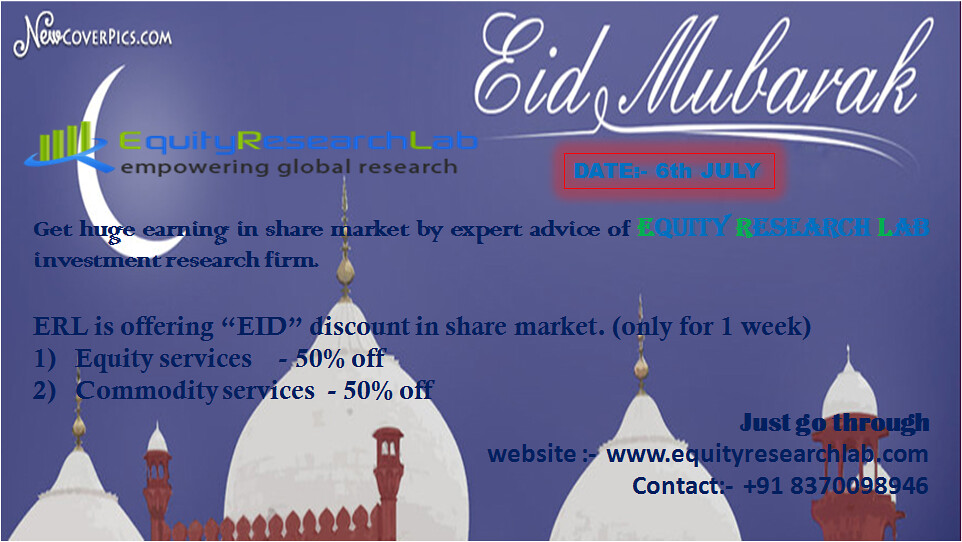The image is an advertisement for Equity Research Lab, dated 6th July, celebrating Eid Mubarak. In the top left corner, it features the company's motto, "Empowering Global Research." The central text promotes a special Eid discount, offering 50% off on both equity and commodity services for one week, with a promise of huge earnings in the share market through expert advice from the Equity Research Lab, an investment research firm (ERL). The contact details and website, www.equityresearchlab.com, along with the phone number +91-837-009-8946, are displayed at the bottom right. The background showcases a deep blue sky with a partial crescent moon and silhouettes of dome towers, giving it a distinctly Middle Eastern appeal.